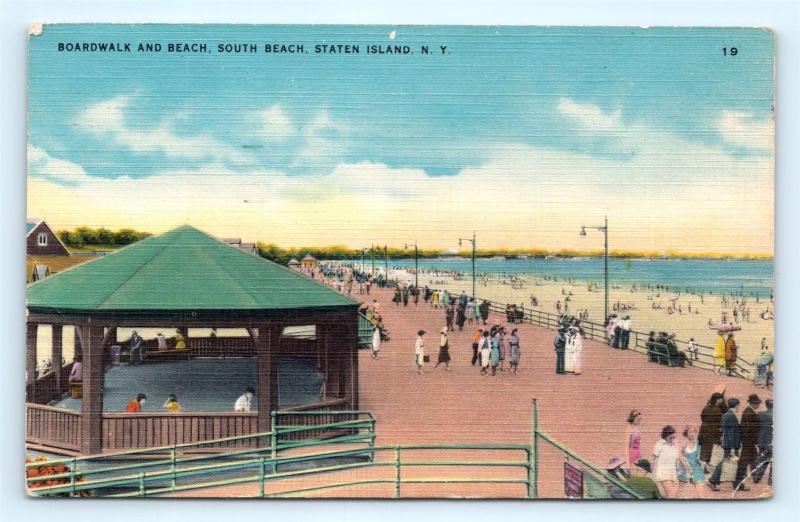The image is a hand-drawn painting capturing a nostalgic scene of "Boardwalk and Beach, South Beach, Staten Island, New York," marked with the number "19" in the top right corner, possibly indicating the year 1919. The left side of the picture features a large green gazebo with a spiraling roof, people seated inside enjoying their time. The boardwalk, reddish-brown in color, stretches across the scene, populated with individuals dressed in a variety of attire, from sundresses to business suits, some even holding colorful parasols. Along the boardwalk’s stretch, more hand-drawn figures, though tiny and obscure, are visible. To the right, the sandy beach leads into the ocean, with a treeline visible in the distance beneath a blue sky dotted with white clouds. In the background, partially obscured, stands a red building with a bluish-gray roof. It's a depiction of a sunny day, with sunlight visible on the horizon, evoking a quaint, early 20th-century seaside atmosphere.